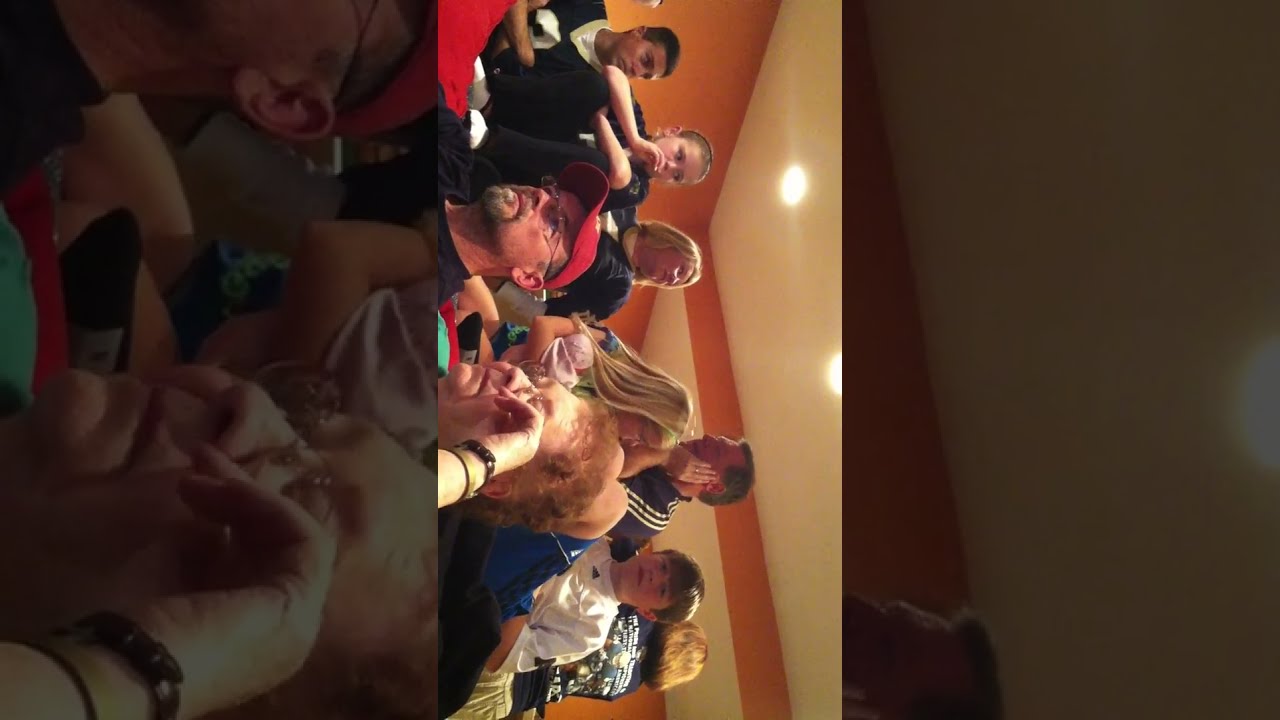The photograph depicts a family gathering indoors, featuring a mix of ages and personalities. The image is rotated 90 degrees, showing a room with bright white walls and ceiling, adorned with soft lighting and hints of orange along the walls. Central to the scene, a young blonde girl, around 9 or 10 years old, is seen wearing glasses, a light green jacket, and a black shirt, looking to her left. In front of her sits an older couple; the man sports a red cap, glasses, a goatee, and a black shirt, while the woman beside him appears to be in her 60s with red curly hair, glasses, and closed eyes, suggesting she might be resting. A middle-aged couple with blonde hair, likely the parents, are situated behind them, smiling warmly. The mother and another daughter, also wearing glasses and blonde, are dressed in black. There's a boy with blonde hair, dressed in blue shorts and a white top, who seems to be eating something. The entire scene suggests a lively, multi-generational family moment.